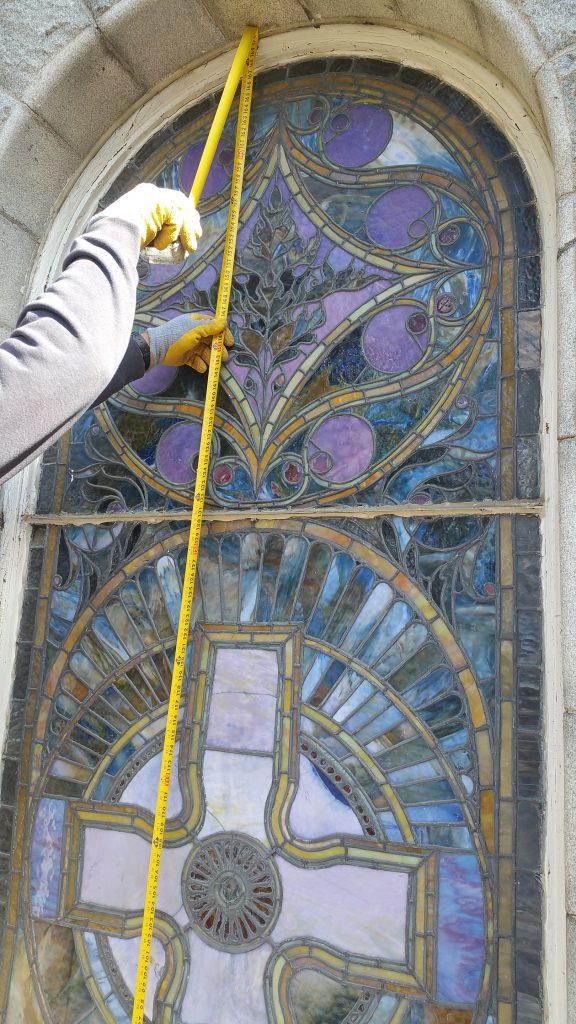A color photograph captures a person, wearing a navy sweatshirt and yellow and gray gloves, using a tape measure to measure the height of a stained glass window. The person’s hands are situated in the upper left corner, and they are utilizing a yellow tape measure. The stained glass window is arched at the top and rectangular at the sides, and it is set within a light gray stone frame embedded in a stone wall.

The stained glass window consists of numerous small, individually stained pieces of glass, featuring a predominantly religious theme. The main section of the window showcases a gold-trimmed cross against a blue background. Above this, the upper part of the window contains a purple diamond, bordered in gold, with a floral or leaf pattern inside, complemented by additional gold and purple circular designs. The stone wall surrounding the window also has sections of yellow paint.